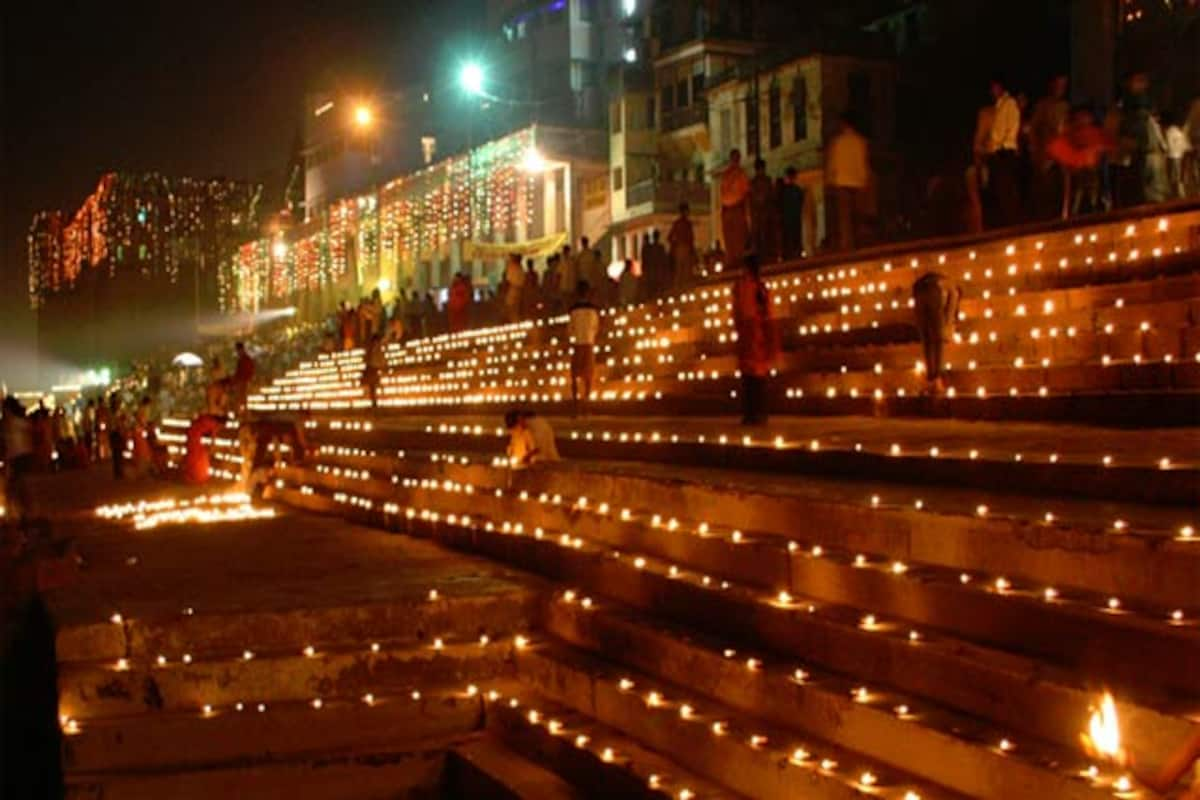This image captures a nighttime candlelit ceremony set on a stepped terrace, reminiscent of scenes from India. The concrete steps, adorned with countless small candles, stretch from the lower right to the middle of the left side of the photograph. Some of the candles have large, flickering flames, while others are smaller, tea light-sized, casting a soft glow over the scene. People, predominantly dark-haired and dressed in non-Western attire, are scattered across the steps, with many gathered at the top and throughout the terrace, participating in or observing the ceremony. Some individuals are seen bending down to light or extinguish the candles. In the background, an urban environment is visible with buildings adorned with string lights and other forms of illumination, enhancing the festive atmosphere. The overall scene is vibrant yet intimate, with the interplay of flames and electric lights creating a warm, serene ambiance.